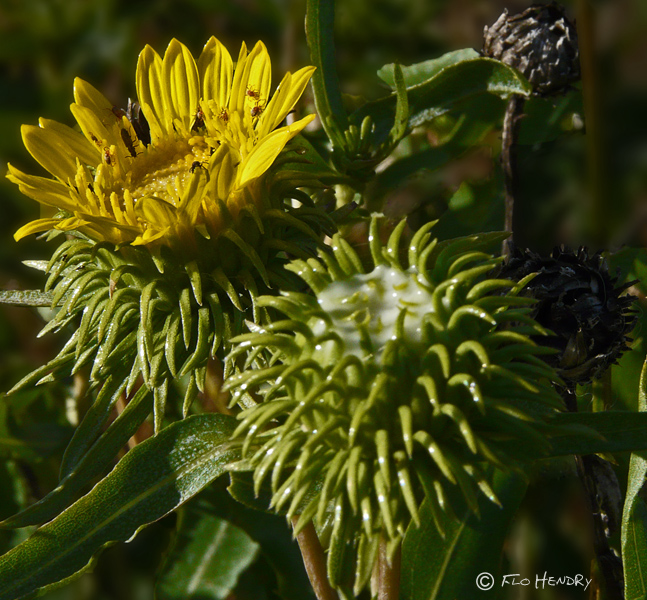In the image, we see a brightly colored yellow daisy-like flower, possibly a Grindelia stricta or gum plant, prominently situated in the upper left-hand corner. This flower is the only one in full bloom and features petals that stick straight up, almost resembling a dandelion. Surrounding the yellow petals are curved, pointed green sepals that lean downward. Accompanying this bloom, there are unbloomed green flower buds with numerous green sprigs extending outward, two of which exhibit a white, possibly milky substance at their centers. Below the main yellow flower and interspersed among the foliage, are wider, broad green leaves and additional green tentacles that add to the plant’s unique appearance. The background of the photo is blurred, composed of muted browns and blues, contributing to the overall focus on the vibrant colors of the gum plant.